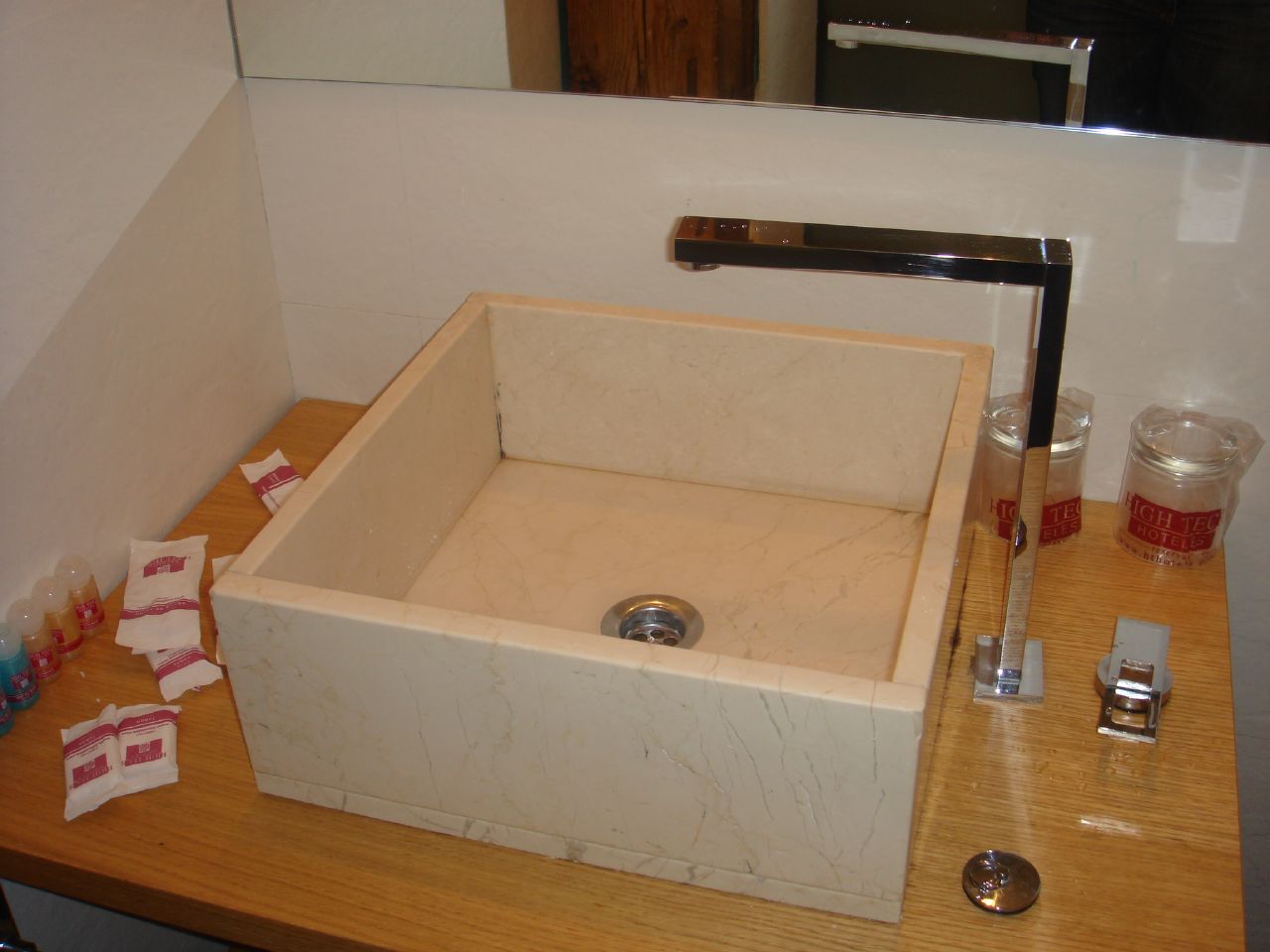The image captures a well-designed bathroom sink area within a horizontal rectangular frame, presenting a realistic photograph. The background consists of a mostly plain white painted wall, typical of a bathroom setting. Surrounding the sink on three sides—left, back, and right—there's a section of slightly off-white tiles approximately 12 inches in height. Above this tiled area, a mirror is affixed, reflecting the sink and faucet below.

The countertop beneath the sink appears to be made of a light brown wood material, with a shiny, stained finish adding a touch of elegance. The sink itself resembles a halved box with dimensions roughly 12 inches by 12 inches, constructed from white marble. It features a stainless steel drain and stands about six inches tall along the edges, creating a modern and sleek design.

The faucet, positioned on the right side of the sink, is constructed from rectangular stainless steel. Its design is minimalist, extending straight up and then across, with a spout directing water downward. A handle for the faucet is located towards the right on the countertop, offering intuitive control.

In the back right corner of the countertop, there are two glass cups wrapped in plastic bags bearing a red label with the phrase "High-Tech Hotels" written in white or transparent letters. On the left side of the sink area, several white bags, possibly containing napkins, are accompanied by transparent bottles adorned with red and green labels, contributing to the organized yet functional aesthetic of the space.